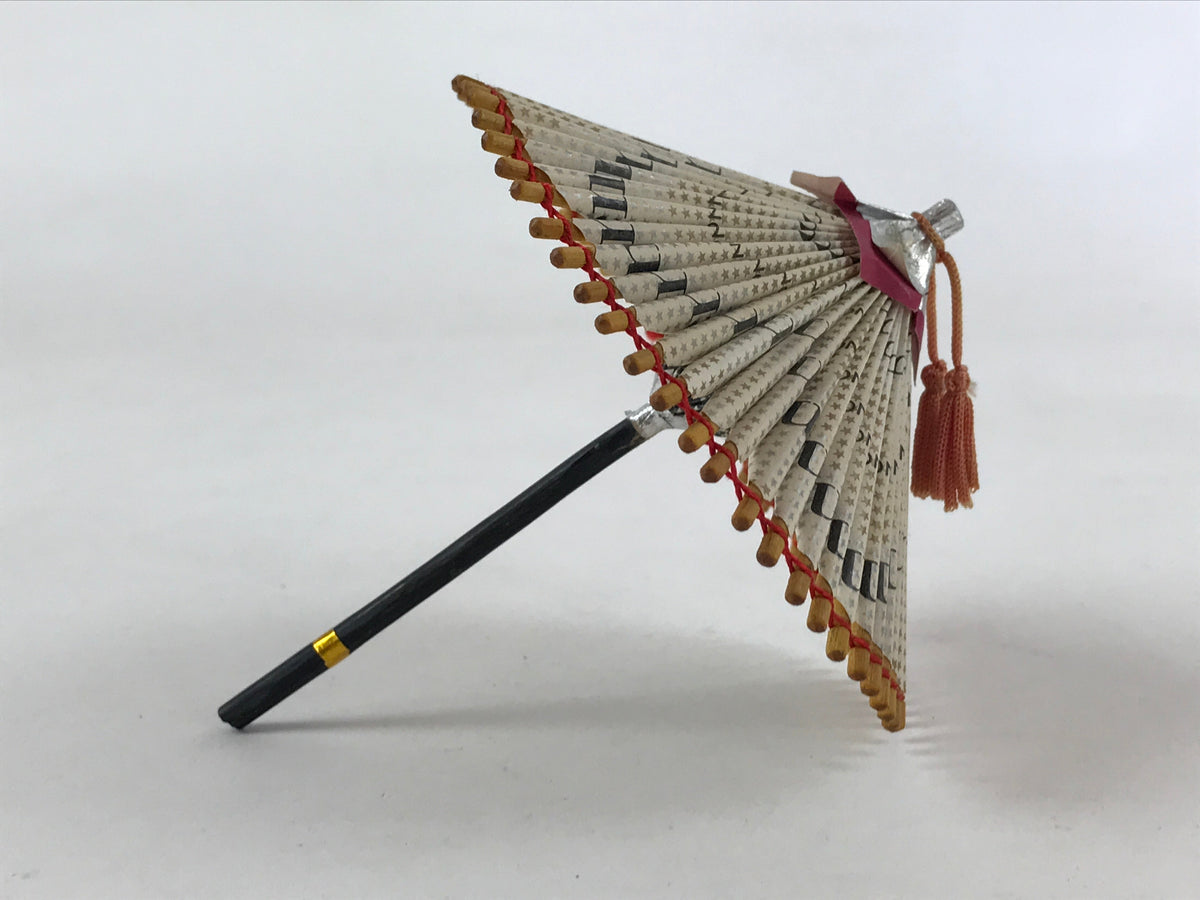This is a detailed professional photograph of what appears to be a museum artifact, a small East Asian parasol or umbrella, likely from Japan and dating from as early as the 1600s to the early 1900s. The artifact is set against a white photography backdrop. The parasol features a straight black handle with gold detailing near its base. The canopy is supported by wooden dowels attached to a silver metal apex, which is adorned with red fabric ruffles and two orange-red tassels tied around the tip. The parasol's cover is a delicate material, possibly fabric or paper, and has an intricate yet indeterminate gold and navy blue pattern, accompanied by black lettering or designs. The detailing around the edges includes an intricate weave of red thread wound around the spokes. From the angle and state of the parasol, it's partially folded, making the designs and any writing not fully visible.